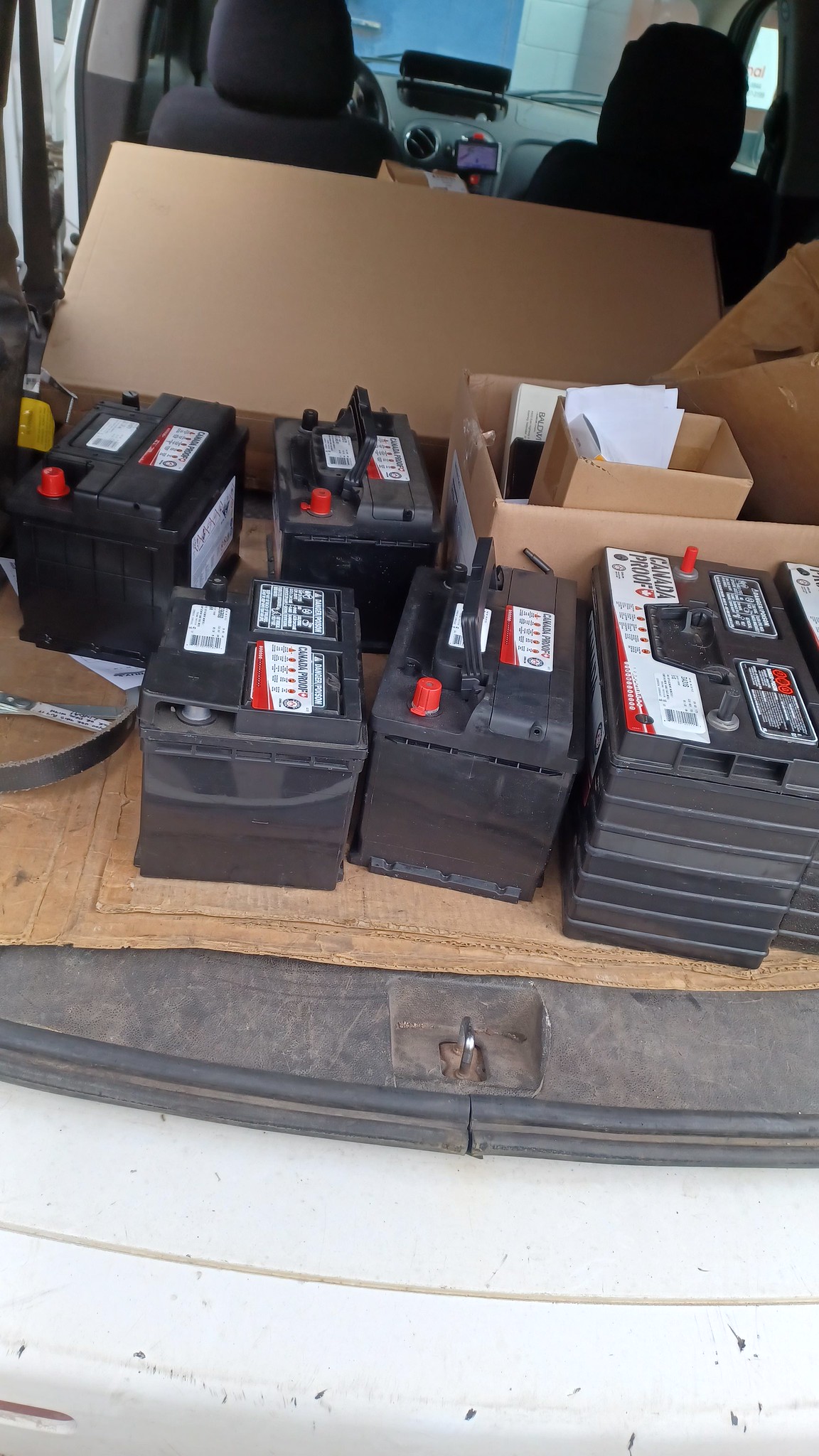This image captures the interior of the back of an SUV or a van, with the rear seats folded down to create an expansive cargo area. Dominating the foreground are six large, black car batteries, with one slightly larger than the others. Each battery features red and black labeling, including some text that reads "Canada Proof," although the complete details of the labels are indistinct. The batteries are neatly arranged on a flattened cardboard box, suggesting careful placement. Surrounding the batteries are additional empty boxes, adding to the sense that these batteries are either being transported for sale or distribution. In the background, the front seats, steering wheel, and a navigation system are visible, confirming the vehicle's interior layout. A trunk latch is also visible, emphasizing the photo's focus on the storage area. The batteries appear to be in good condition, further implying their commercial intent rather than disposal.